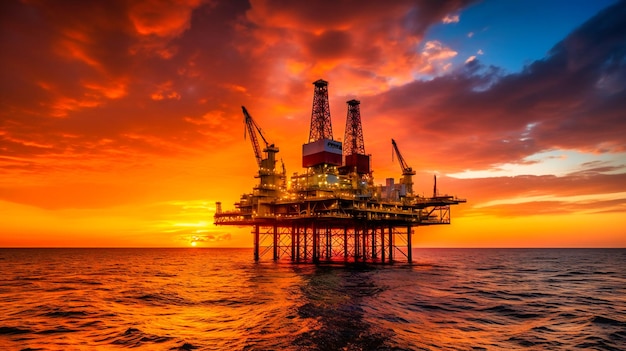The image depicts an oil platform set against a dramatic ocean sunset. The sun is very low on the horizon, casting a vibrant palette of orange, yellow, and red across the sky, with a small patch of blue peeking through in the top-right corner. The reflective waters below adopt these warm hues, appearing somewhat choppy yet not tumultuous. The rig itself, elevated on formidable steel stilts, boasts a complex structure with multiple levels and an array of cranes and towers rising prominently from its center. White lights illuminate various parts of the platform, suggesting activity, though no specific details or workers are visible from this distance. The sprawling metal supports of the rig frame visible portions of both sea and sky, encapsulating the industrial might against a serene yet vivid natural canvas.